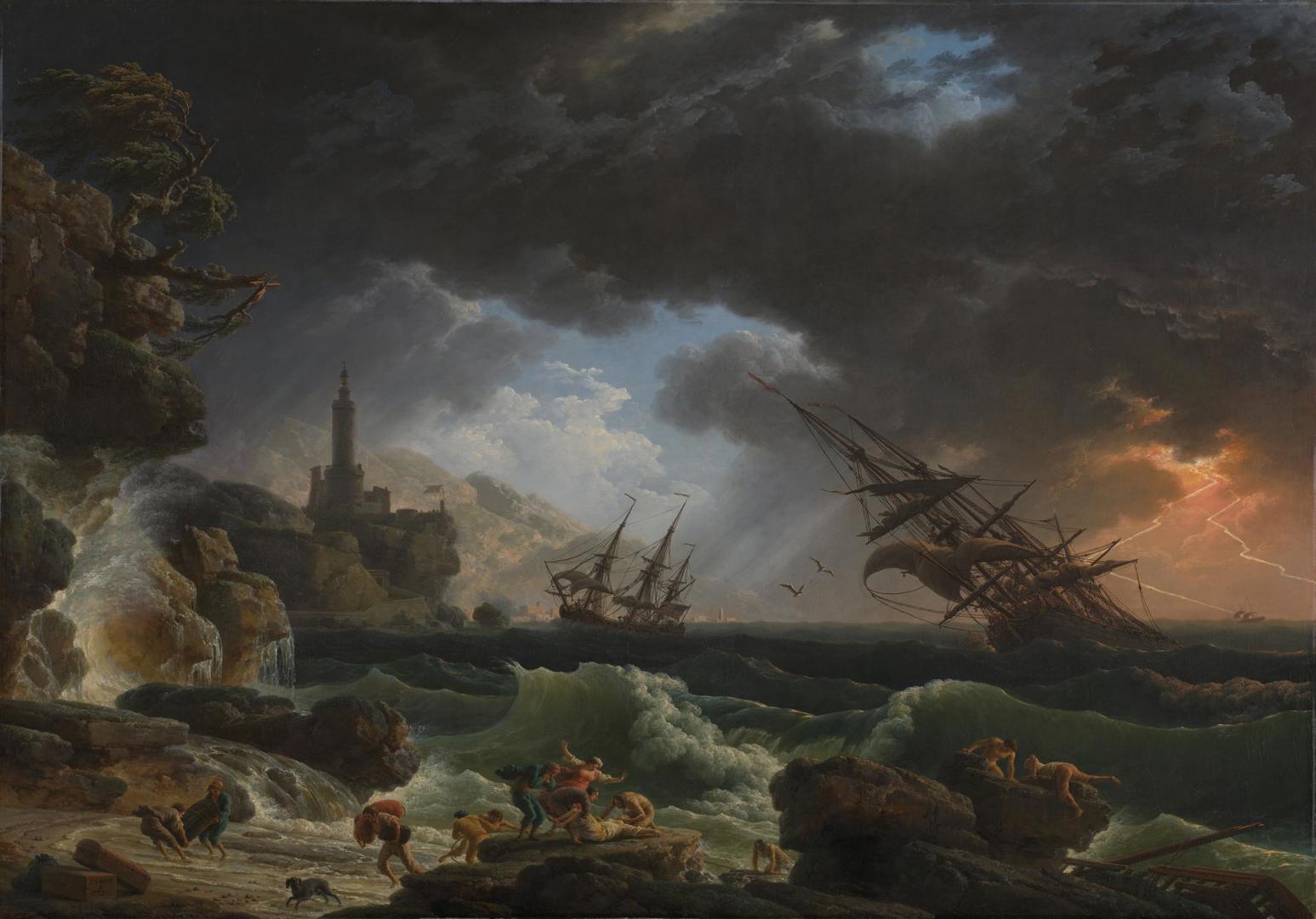This horizontally aligned, almost square-shaped artwork presents a tumultuous and dramatic seascape dominated by a stormy sky. The upper portion of the image features an angry-looking sky filled with black, fluffy clouds occasionally interspersed with patches of white and hints of blue breaking through. Diagonal streaks of gray suggest heavy rain, while vibrant yellow lightning bolts slice through a mix of orangish-gray clouds on the right side.

Beneath this turbulent sky stretches a rough, churning ocean, its dark, rough water almost seeming to battle the small wooden sailboats caught within it. The two brown sailboats, tilted precariously, highlight the ferocity of the storm; one is centrally located while the other is to the right. The water's violent motion underscores their struggle against the elements.

In the foreground, crashing waves threaten a rocky shoreline on the left. Here, amidst the chaos, human figures appear, seemingly running for cover or attempting to swim ashore. To the far left, built into a cliffside, stands what appears to be a castle, its spire rising ominously against the stormy background. The meticulous details of this painting, from the storm-tossed boats to the fleeing individuals, capture a moment of intense natural drama, reminiscent of historical art pieces found in renowned museums.